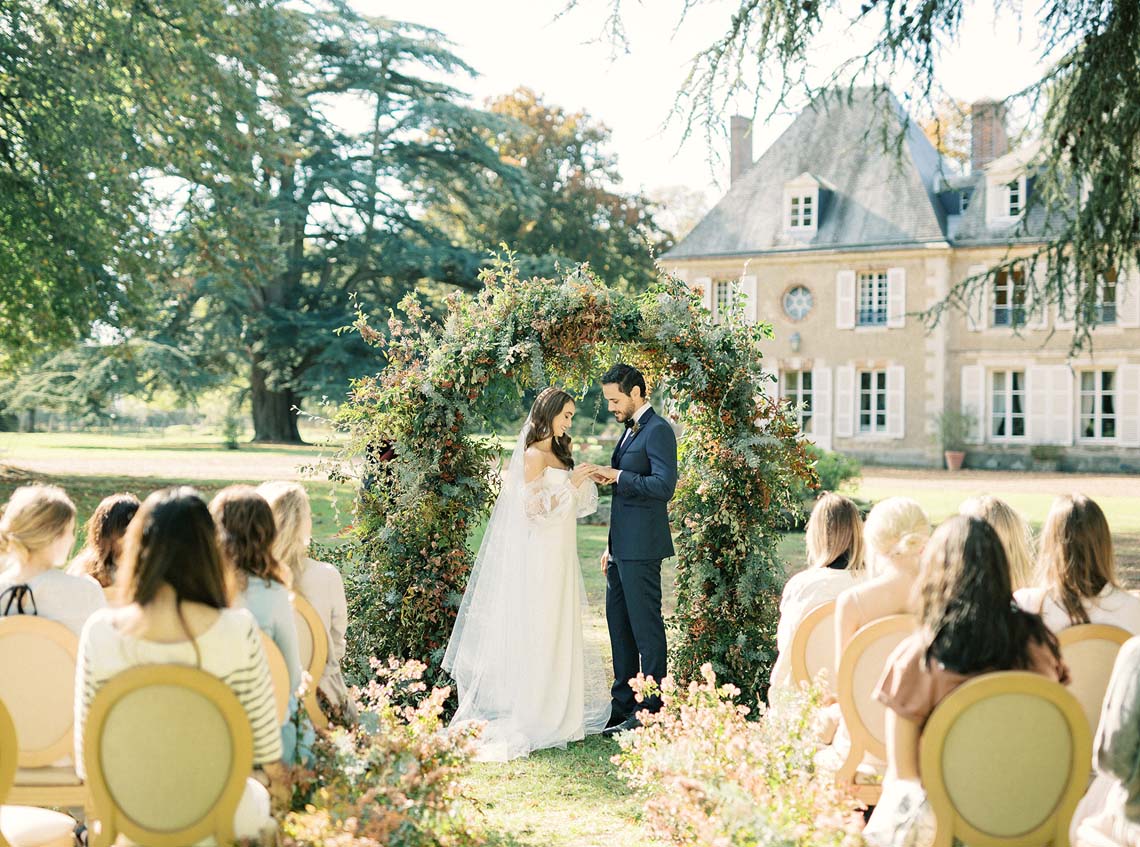This horizontal rectangular photograph captures an outdoor wedding ceremony set against the backdrop of a large, yellow mansion with concrete block corners, steep roof, and dormer windows. In the foreground, the bride and groom stand under a leafy arch adorned with fall-colored leaves, appearing to exchange wedding rings. The bride, wearing an off-the-shoulder long gown with a chiffon overskirt, lace sleeves, and a long, trailing veil, faces the groom dressed in a dark gray suit with black lapels, a flower on his lapel, a white undershirt, and a black bow tie. Guests, viewed from behind, are seated in oval-backed wooden framed chairs arranged in two rows along a grassy aisle adorned with green plants and flowers. The audience includes women in a variety of colorful dresses, adding to the lively and vibrant atmosphere of the celebration. Beyond the arch, the mansion's tan brickwork and white-trimmed windows, amid green and brown trees, complete the picturesque scene.